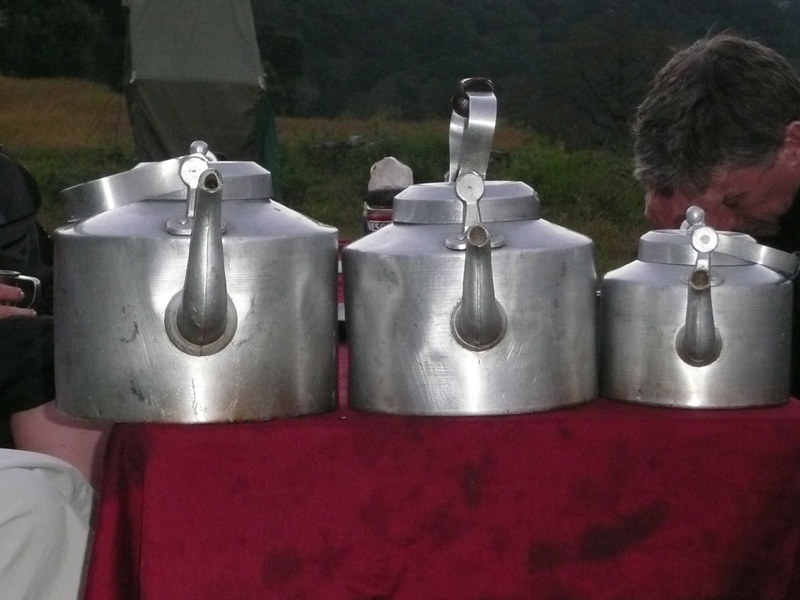The photograph depicts a colorful, outdoor setting with a predominately landscape orientation. Dominating the foreground is a weathered red, almost maroon, tablecloth, marked with dark splotches indicating prolonged use without washing. Atop this tablecloth sits a series of three bulky, polished steel or aluminum kettles arranged from left to right in descending size. Each kettle features prominent spouts and gauges, suggesting they could either be teapots or pressure cookers, with large circular handles equipped with grips at the top. The spouts are all facing towards the camera, emphasizing their utilitarian design.

To the right of the kettles, a man with dark brown hair rests his forehead in his hand, possibly in contemplation or fatigue. Partially visible on the far right side of the image are the lower limbs of two other individuals; one appears to be wearing a skirt while the other is in long pants, suggesting a mixed-gender group. The setting exudes a rural charm, reinforced by the backdrop of tall, green and yellow grasses and scattered trees, evoking the ambiance of an estate sale or a quaint, country market stall.